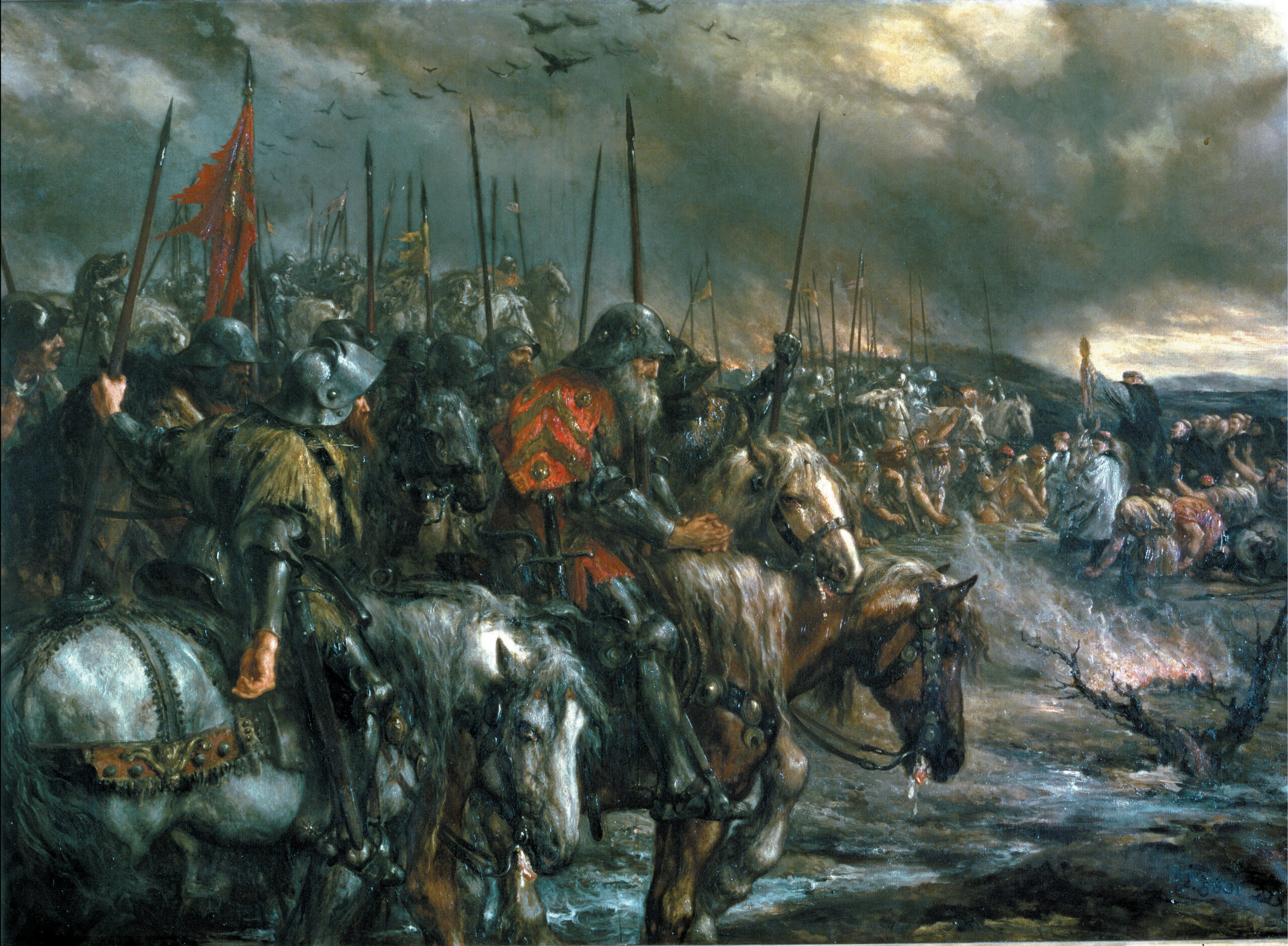This detailed oil painting captures the ominous start of an ancient battle, presenting a vertical rectangular composition. The top of the image is dominated by a stormy sky, with dark, gray clouds pierced by slivers of light on one side, and silhouettes of black birds flying overhead. Below, a line of weary-looking mounted warriors stretches from the left all the way to the right center, their horses appearing fatigued. The soldiers wear old, gray metal helmets, with various pieces of armor and cloth around their shoulders, and they clutch large wooden staffs or pikes. At the forefront rides a man on a gray horse with a prominent long gray beard, possibly the leader, distinguished by red shoulder pads adorned with gold triangles. The ground beneath them is dark and grim, resembling a burnt battlefield. To the right, in front of the horses, rows of people sit or bow, perhaps prisoners or those praying amidst the grim scene. The overall palette consists of somber colors: grays, blacks, reds, yellows, off-whites, browns, light browns, tans, and beiges, emphasizing the bleak and grim atmosphere of the impending battle.